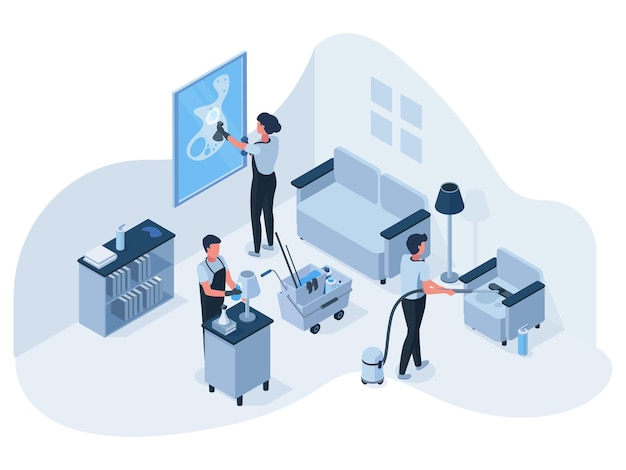This detailed cartoon drawing depicts a cleaning scene in a living room setting, viewed from a top-down perspective. Three individuals, possibly janitors or maids, are engaged in cleaning various parts of the room. The color palette of the image consists of light pastel blues, whites, and blacks, lending a simplistic yet charming aesthetic.

On the right side, a man with black hair, dressed in white with black pants, is vacuuming or steam-cleaning a small armchair using a long black tube attached to a silver canister. Next to him, a woman in the middle of the scene, wearing an apron over a blue t-shirt, is meticulously wiping down a lamp that sits on a small table. Also at the center is a silver cart equipped with cleaning supplies, including mops and a bucket of water.

To the left, another woman is cleaning the glass on a portrait hanging on the wall to make it shine. Additional furniture includes a blocky couch and bookshelf, further detailing the room. All three cleaners share a similar Hispanic appearance and are outfitted in coordinated cleaning attire. The overall composition of the room features blocky, simple furniture designs, enhancing the minimalistic yet engaging visual appeal of the drawing.